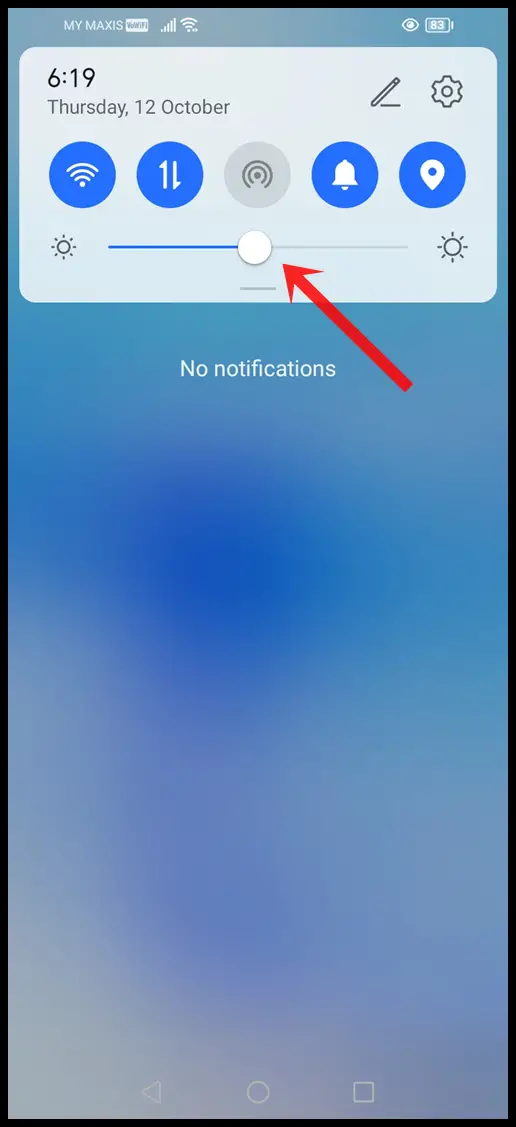This image is a screenshot taken from a cell phone in portrait mode. In the upper left-hand corner, the status bar displays the text "my Maxis Maxis" along with an icon labeled "Vo Wi-Fi." The upper right-hand corner of the status bar shows a battery icon indicating 83% charge. 

The background of the screenshot is an abstract wallpaper featuring shades of dark blue, light blue, and light cream. At the top of the screen, there is a light gray rectangular box with rounded corners, displaying the time as "6:19" and the date as "Thursday, 12th of October." In the upper right corner of this box, there is an icon that allows you to edit the display.

Below the time and date box, five blue icons are arranged horizontally. The middle icon, representing Wi-Fi, is gray suggesting that it is currently inactive. 

Further down, there is a brightness adjustment slider. Moving the slider to the left darkens the screen, while moving it to the right brightens the screen; currently, the slider is centered. A red arrow points to this slider, helping users easily locate the brightness control function. At the very bottom of the screen, text reads "No notifications," indicating that there are no current alerts or messages.